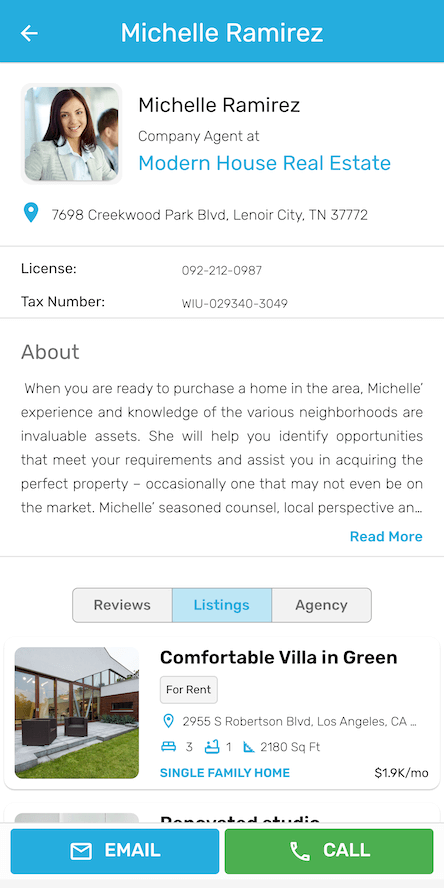The image depicts a phone interface in portrait mode featuring the profile of Michelle Ramirez, a company agent at Modern House Real Estate. At the top of the screen, there's a blue header with white text reading "Michelle Ramirez" accompanied by a left-pointing white arrow. Below that, in a white section, her name appears again in black text.

To the left of her name, there's a small box displaying her picture where she is smiling at the camera, dressed in professional attire. Her title, "Company Agent at Modern House Real Estate," is written below her name in blue text. Further down, the screen lists her address as 7698 Creekwood Park Boulevard, Lenoir City, Tennessee 37772, followed by her license number, 092-212-0987, and a tax number.

The next section contains a brief description stating: "When you're ready to purchase a home in the area, Michelle's experience and knowledge of the various neighborhoods are invaluable assets," indicating her expertise and offering more details about her services.

At the bottom of the screen, there are three tabs: Reviews, Listings, and Agency, with the Listings tab highlighted. The Listings tab features information about a property titled "Comfortable Villa" in green and black text, showing an image of the villa's exterior with outdoor seating and a lawn. The property is categorized as a single-family home. Two buttons are present at the bottom of the listing: one in blue labeled "Email" and the other in green labeled "Call."